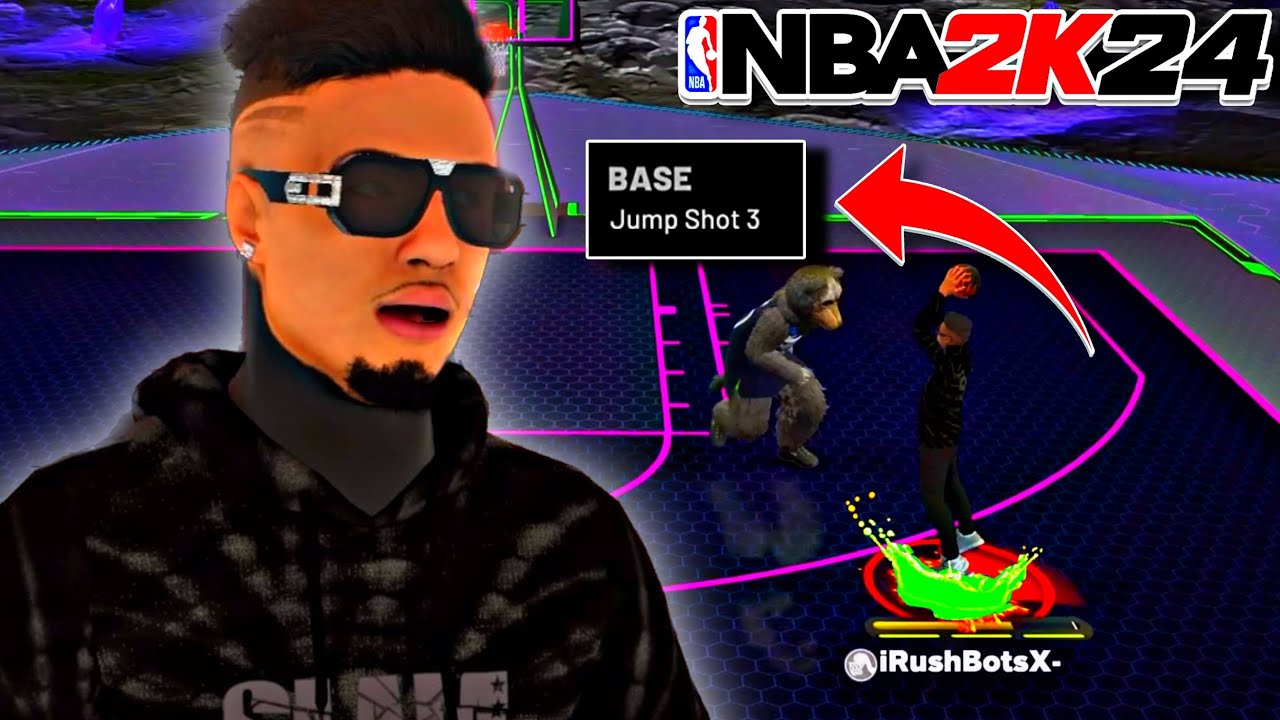In the screenshot from the highly realistic game, a darker-skinned avatar is prominently displayed on the left side of the screen. The avatar, resembling a gentleman, sports black sunglasses adorned with diamond detailing. He has short black hair, faded on the sides, and a small goatee beneath his lower lip. His mouth is slightly open, giving him an expressive appearance. He is dressed in a black hoodie with subtle gray accents.

Positioned in the top right corner, the NBA logo is visible, accompanied by the text "NBA" in black, "2K" in red, and the number "24" in black lettering. Below the logo, there is a left-curving arrow next to a black rectangle with a white border, displaying the text "Base Jump Shot 3."

Additionally, the image includes two distinct characters at the bottom. One appears to be a brown, S-shaped, monster-like creature with a duck bill. The other character resembles a monster as well but is more humanized, holding a basketball, dressed in all black with white tennis shoes, and sporting short cropped hair. A green blotch and a red circle are beneath these characters, and below them, in white text, is the username "irishbotsx."